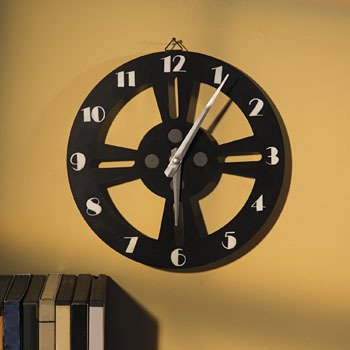The image depicts a black clock mounted on a wall painted in a rich golden ochre color. The clock features stark white hands, indicating the time as approximately 6:06. Surrounding the clock face are white numerals, providing clear contrast against the black. At the center of the clock is a distinctive cross-shaped design, with cutout sections interspersed between the arms of the cross, adding an element of visual intrigue. In the bottom left corner of the image, a neat stack of books rests against the ochre wall, providing an additional layer of interest to the composition.